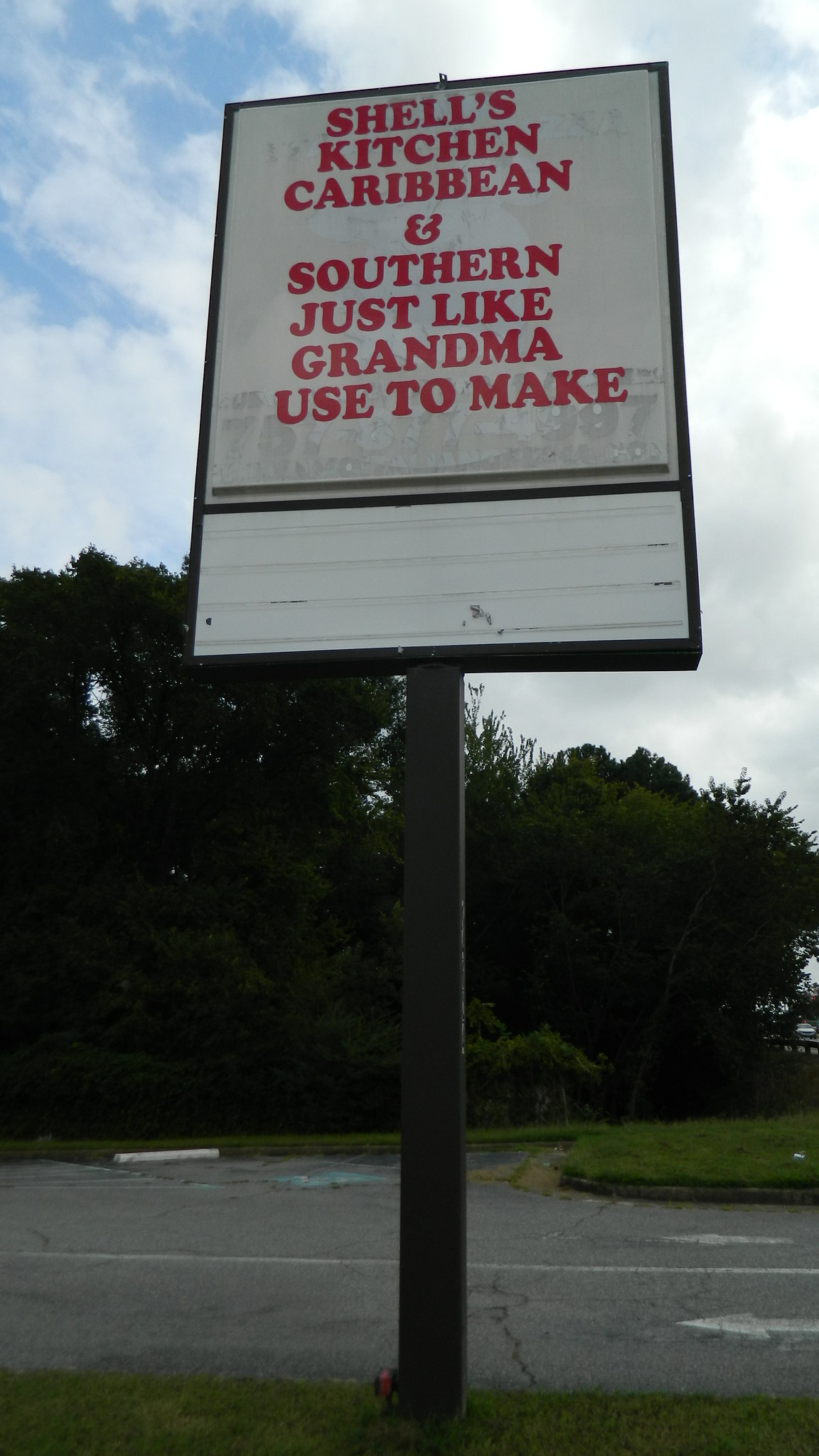The image is a tall, portrait-oriented, outdoor color photograph dominated by a large, rectangular sign mounted on a thick, rectangular, metal pole that extends vertically from a grassy verge. The sign, positioned in the top third of the image, has a white background with a black border and features red text spread across multiple lines: "Shell's Kitchen, Caribbean and Southern, just like Grandma used to make." The worn remnants of old signage are faintly visible beneath the current letters.

In the foreground, we see green grass at the base of the pole. Behind the sign and stretching into the background is a grey asphalt road, featuring part of an arrow and a white lane divider. Across the road lies another strip of grass, leading to a small wooded area with tall, dark trees that are slightly underexposed. Above the sign, the sky is predominantly cloudy, with a small patch of blue visible in the top left corner. The text's nostalgic phrase suggests the sign is advertising a North American eatery specializing in Caribbean and Southern cuisine.